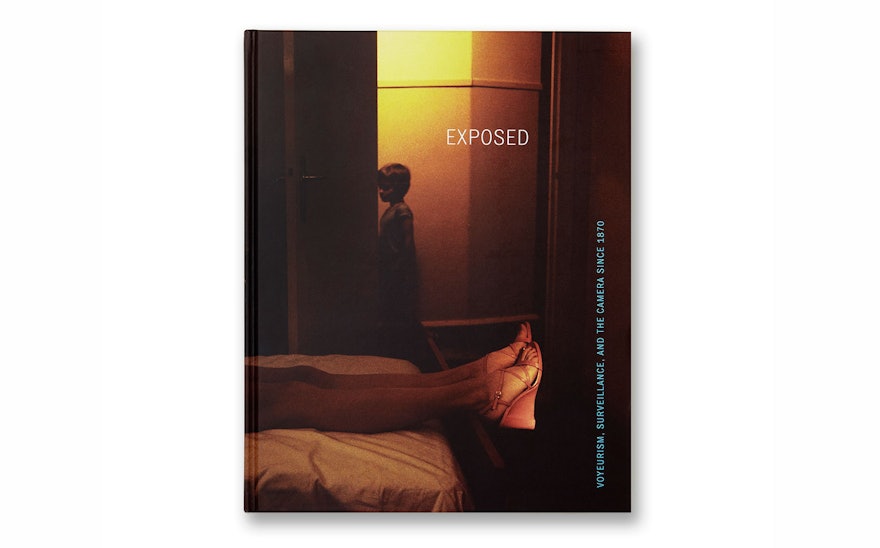The image appears to be the cover of a documentary, dominated by a warm, eerie golden light that creates an unsettling atmosphere. The scene captures a softly lit bedroom with white sheets, where a woman in strappy pink wedge heels lies on a bed, her legs hanging off the edge. To the right side of the image, text in light blue capital letters reads, "voyeurism, surveillance, and the camera since 1870," stretching vertically from the bottom right to the midpoint of the image. Above this, closer to the top right, another piece of text states "EXPOSED" in large, bold letters. The background includes yellow and white walls with wooden elements, adding to the scene’s vintage feel. In the hallway outside the bedroom door, a young boy in a green short-sleeved shirt with brown hair walks by, appearing eerily ghost-like. The overall composition, punctuated by warm orange lighting from the top right corner, reinforces the image's mysterious and voyeuristic vibe.